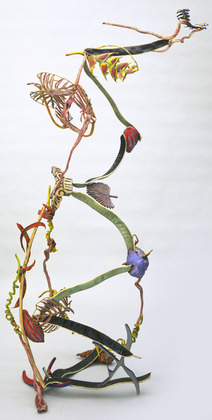The image depicts a complex and abstract sculpture featuring a variety of materials, evoking a blend of natural and minimalist aesthetics. The sculpture is anchored by a triangular base with three potted sections, two of which are green and appear to be metal. Ascending from this base is a chaotic yet intriguing network of elements, including twisted twigs, dried vegetative material, and metal branches. A prominent brown branch on the left and another branch with greenish twigs extend upward, contributing to the sculpture's organic feel. Interspersed within this arrangement are green bean-like shapes and a striking red component. The piece showcases a variety of colors and textures, including a blue nut-like object that serves as a joint, and a lavender rock integrated into the structure. A singular curly stem or wire rises towards the top, crowned by what looks like a curly, brown flower or perhaps bark. The design of the sculpture is sparse, yet rich in details, reminiscent of a Picasso painting in its abstract form.